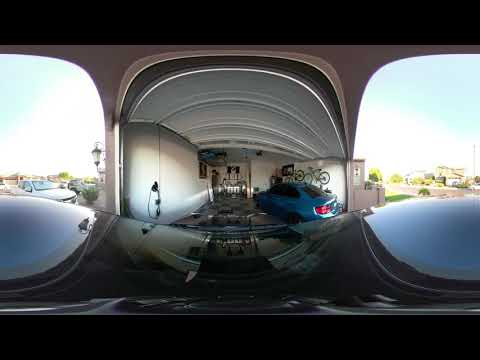This panoramic image, taken from the perspective of a dash camera, captures the interior of a garage with considerable distortion, stretching the scene into a circular shape. Central to the image is a blue sedan parked inside the garage. Mounted on the wall behind the car are two bicycles, along with assorted wires and hoses. The camera is situated on the reflective black hood of another vehicle, adding to the unusual warped effect. The garage's interior walls are white and hold various equipment. The edges of the panorama, which appear as two separate panels due to the distortion, show the garage entryway with a bright blue sky outside. To the left, there are cars parked outside, while on the right, there is at least one building and some trees. This mixed indoor and outdoor view contributes to the disorienting nature of the image, making it challenging to discern whether the garage belongs to a residence or a business.